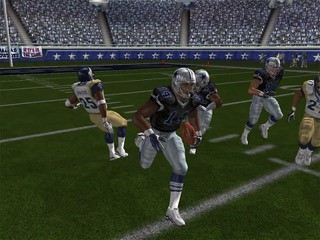The image appears to be an AI or computer-generated graphic, likely taken from a video game. It depicts a vibrant football field with lush green grass and clearly defined white markings for different field zones. The background features a tightly packed audience, represented as tiny dots, watching the game intently from behind a long, blue wall that is adorned with star-like embellishments. 

In the foreground, five players are in dynamic action. One player is prominently captured in mid-stride, clutching the football, with one leg in the air, poised for his next step. Another player appears to have abruptly halted, perhaps realizing he wouldn’t be able to intercept the ball. The remaining players are depicted mid-stride, seemingly in hot pursuit of the ball carrier, each frozen in a moment of intense action. The scene conveys a sense of urgency and athleticism, characteristic of a high-stakes moment in a football game.